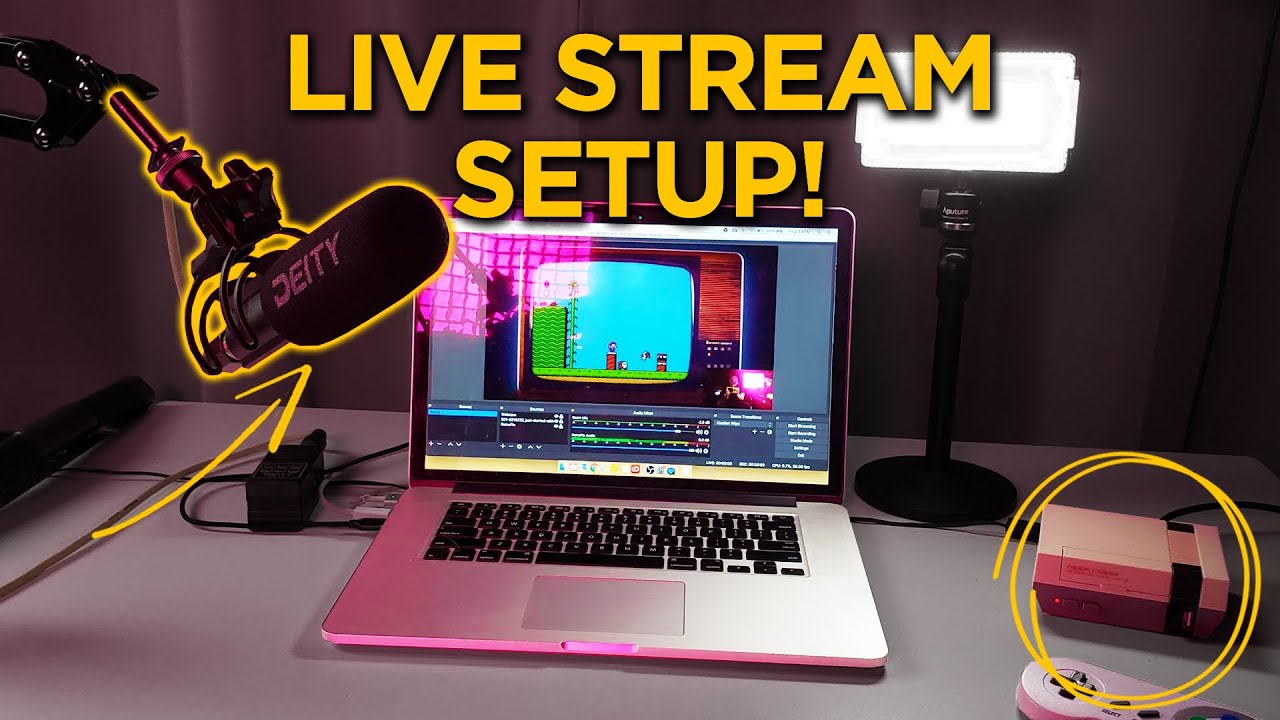This image depicts a detailed live streaming setup on a light gray desk with a gray background wall. Central to the setup is an open pink MacBook displaying a Super Mario game emulator. To its immediate right stands a bright white LED light and further right, a Nintendo electronic system with a controller attached. To the left of the laptop is a hardware dock equipped with switches. Also on the left, a prominent microphone labeled "DADY" in white letters and accentuated with a yellow outline, highlighted by a yellow arrow, draws attention. The top center of the image features the yellow caption "Live Stream Setup!" This elaborate arrangement of streaming equipment is indicative of a YouTube thumbnail setup, designed to showcase the components of a professional gaming live stream environment.